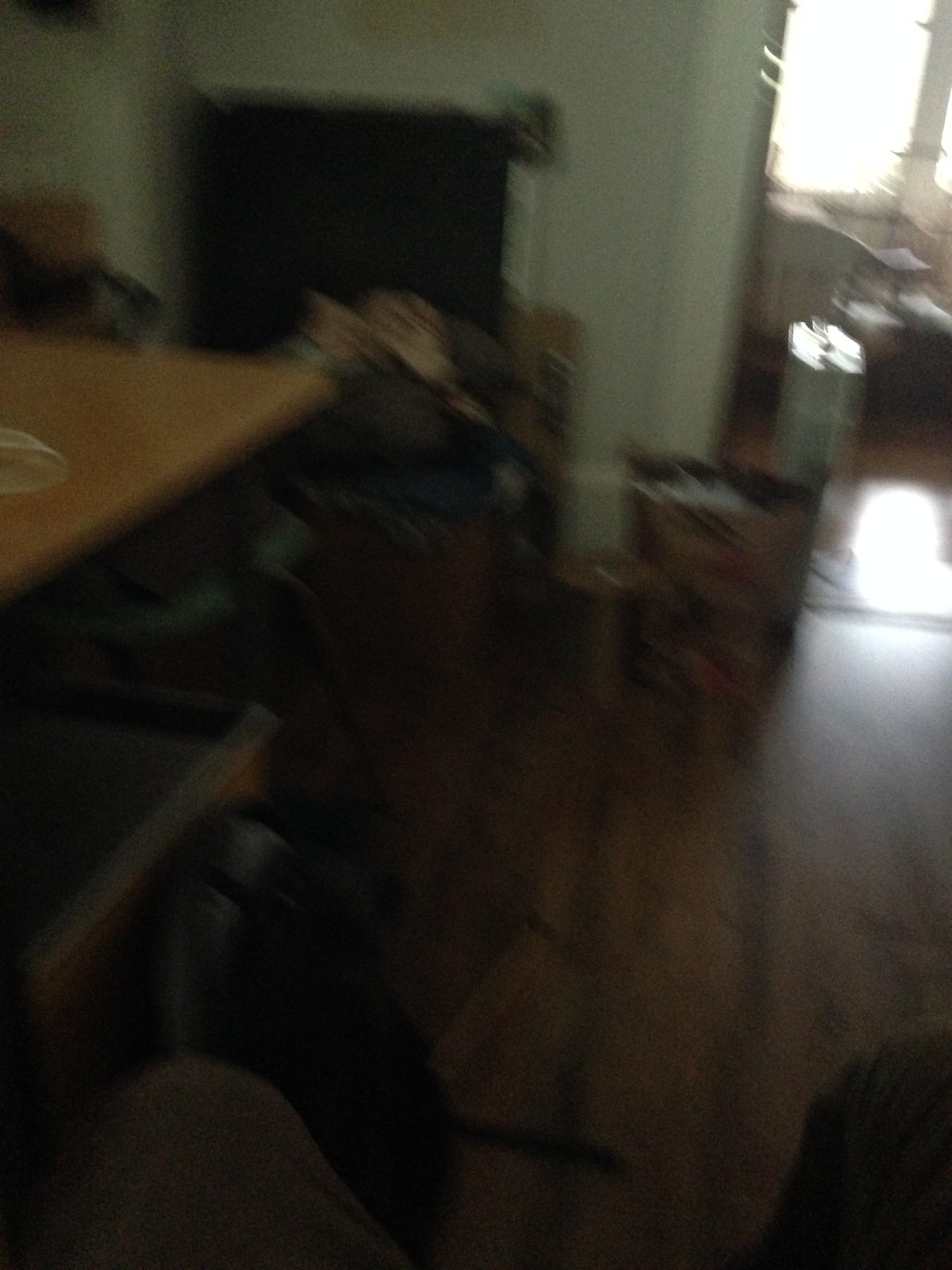In this very blurry image taken inside a home, the foreground is dominated by someone's knees, which are slightly apart and clad in tan pants. The knees are positioned, one in the right-hand corner and the other nearly to the left-hand corner of the frame. On the left side of the image, a brown-topped desk is faintly visible, accompanied by what appears to be a chair, though both are obscured by the blur. The background reveals a white wall covering half of the image, with what looks like a TV screen placed in front of it. Further to the left, a doorway opens into another room, which is illuminated by light streaming through a window. The flooring in the foreground is dark wood, contrasting with a lighter floor visible in the adjoining room.